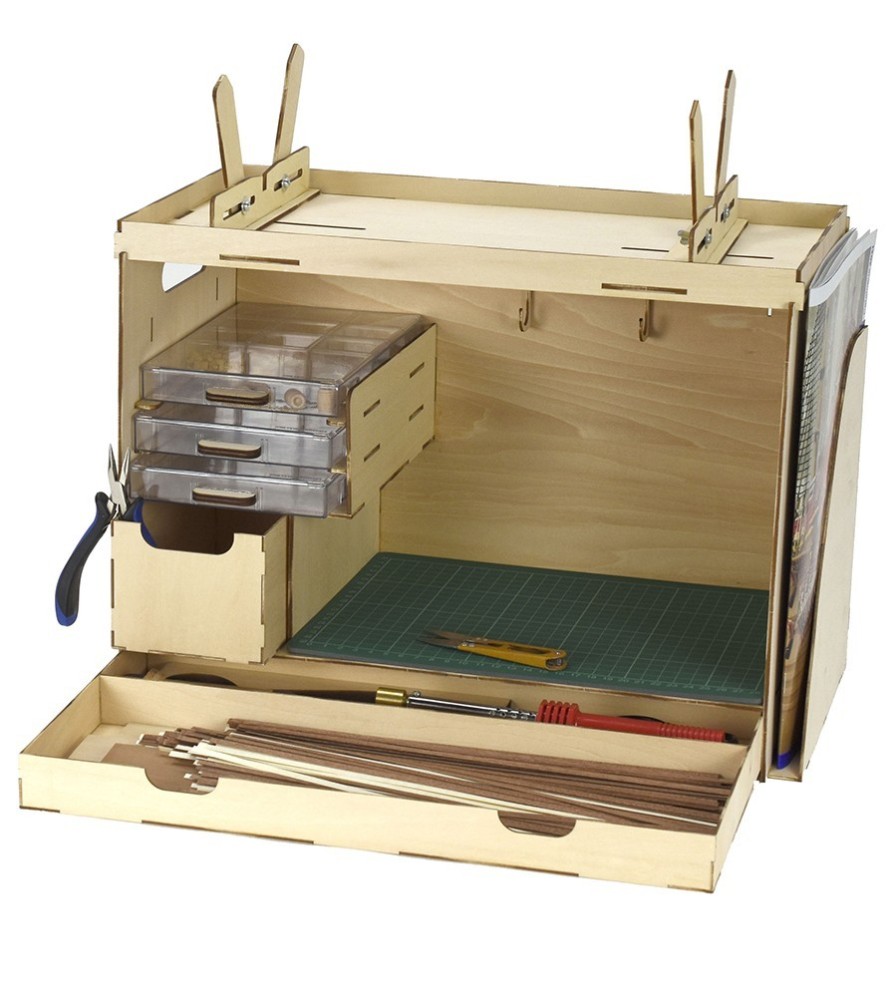This detailed model of the British ship HMS Supply showcases a highly intricate design. The ship, predominantly brown with black and yellow stripes along the side and a blue stripe near the stern, is mounted on a black display stand that is trapezoidal from the front and back, yet rectangular from the side views. A gold faceplate on the stand prominently reads "HMS Supply." The vessel is adorned with numerous white sails, rigged with intricate ropes and positioned between tall masts. A noteworthy feature is the array of flags: a current British flag on a prominent pole extending from the bow, a historic British ensign at the stern with a solid blue field and a Union Jack in the upper corner, and atop the tallest mast, a triangular flag with a Swiss flag design at the hoist followed by red, white, and blue stripes.

The meticulous attention to detail continues with the miniature crew members scattered across the deck. Most of these figures are dressed in blue coats and white pants, while a few are in different colored outfits including yellow shirts with blue pants and vice versa. Additionally, the ship includes a small white lifeboat trimmed in black and blue. The deck is adorned with nets and other fine details, contributing to the authenticity of the model. Overall, this model delivers a rich and accurate portrayal of the HMS Supply, ideal for historical display.